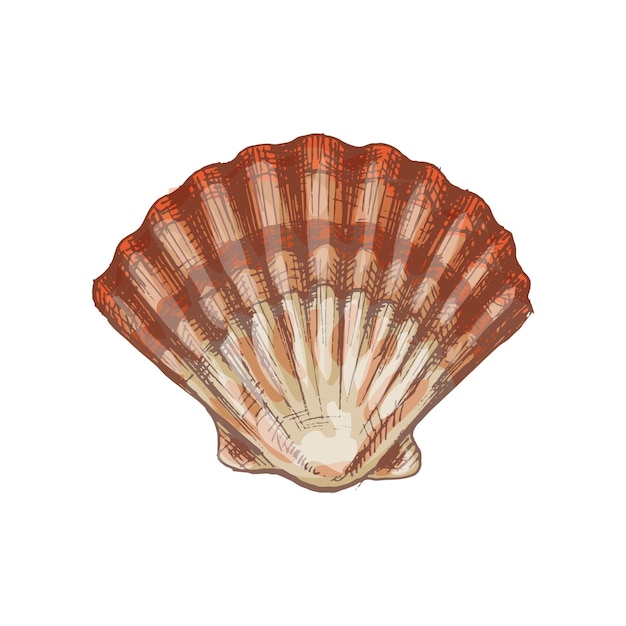This is a detailed animated illustration of a clam shell positioned upright on a white background. The shell features a distinctive red and off-white or beige color scheme with multiple indentations and folds that fan out from the bottom to the top. The drawing uses black ink for the outlines and dark brown lines that resemble hash marks, giving it a highly detailed and reflective appearance. The top of the shell has a vibrant strip of red-orange followed by a sequence of lighter and darker orange sections, transitioning to a lighter area beneath. The lower portion showcases a mix of light brown, white, and very light pink hues, all accented with dark brown and white highlights, enhancing its reflective, almost plastic-like look. The fan-shaped shell captures a gradient of colors from pinks to oranges and reds, making it a striking and beautiful depiction.